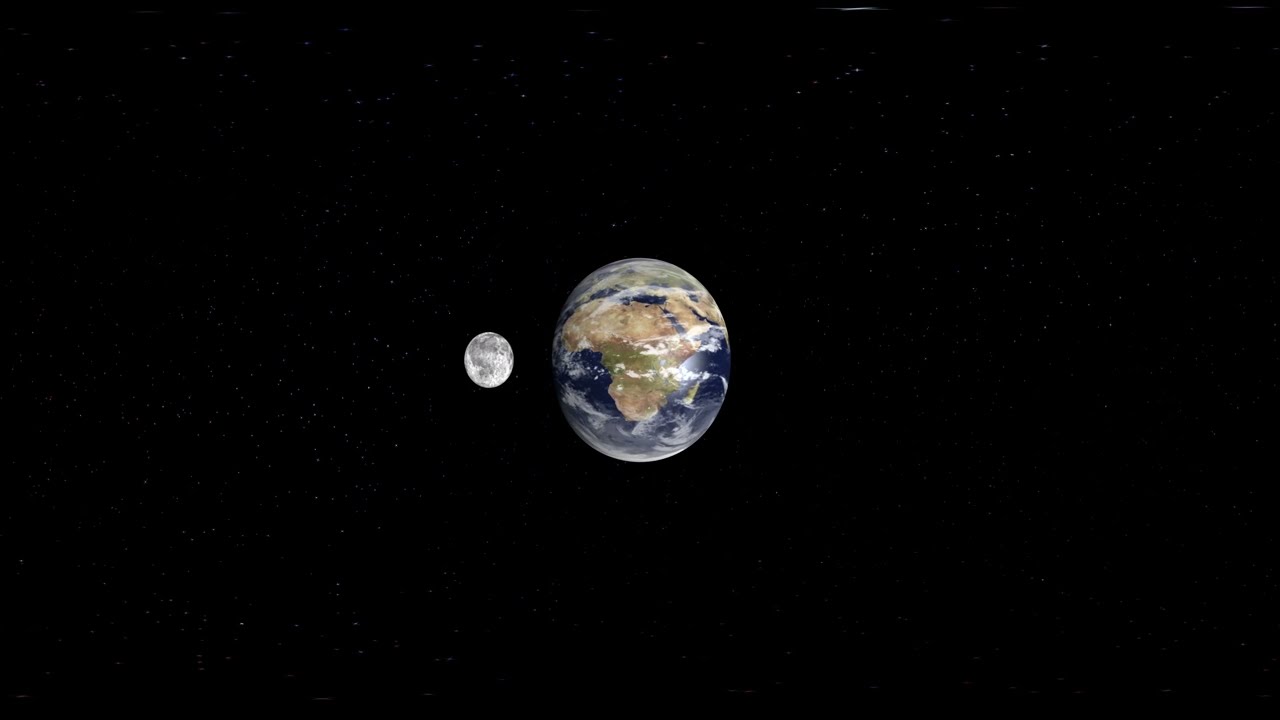The image is a meticulously crafted digital rendering of the Earth from orbit, featuring precise details and high resolution, capturing a vividly sunlit view. The Earth appears slightly elliptical, elongated upwards and compressed from the sides. Dominating the center is the vibrant blue of the Indian Ocean, with the entire continent of Africa, the Arabian Peninsula, and regions extending towards the Near East and India clearly visible, while the northern parts of these regions are partially obscured by clouds. Streaks of clouds are scattered across the planet, yet large areas of land and ocean remain unobstructed. Positioned to the left of Earth is the moon, appearing significantly smaller, about a 20th of Earth's size, with roughly an eighth of its surface obscured by Earth's edge. The moon's surface presents a white with grayish-black specks. The background of the image is a profound black, sprinkled with small bright specks representing distant stars, enhancing the cosmic tranquility of the scene.